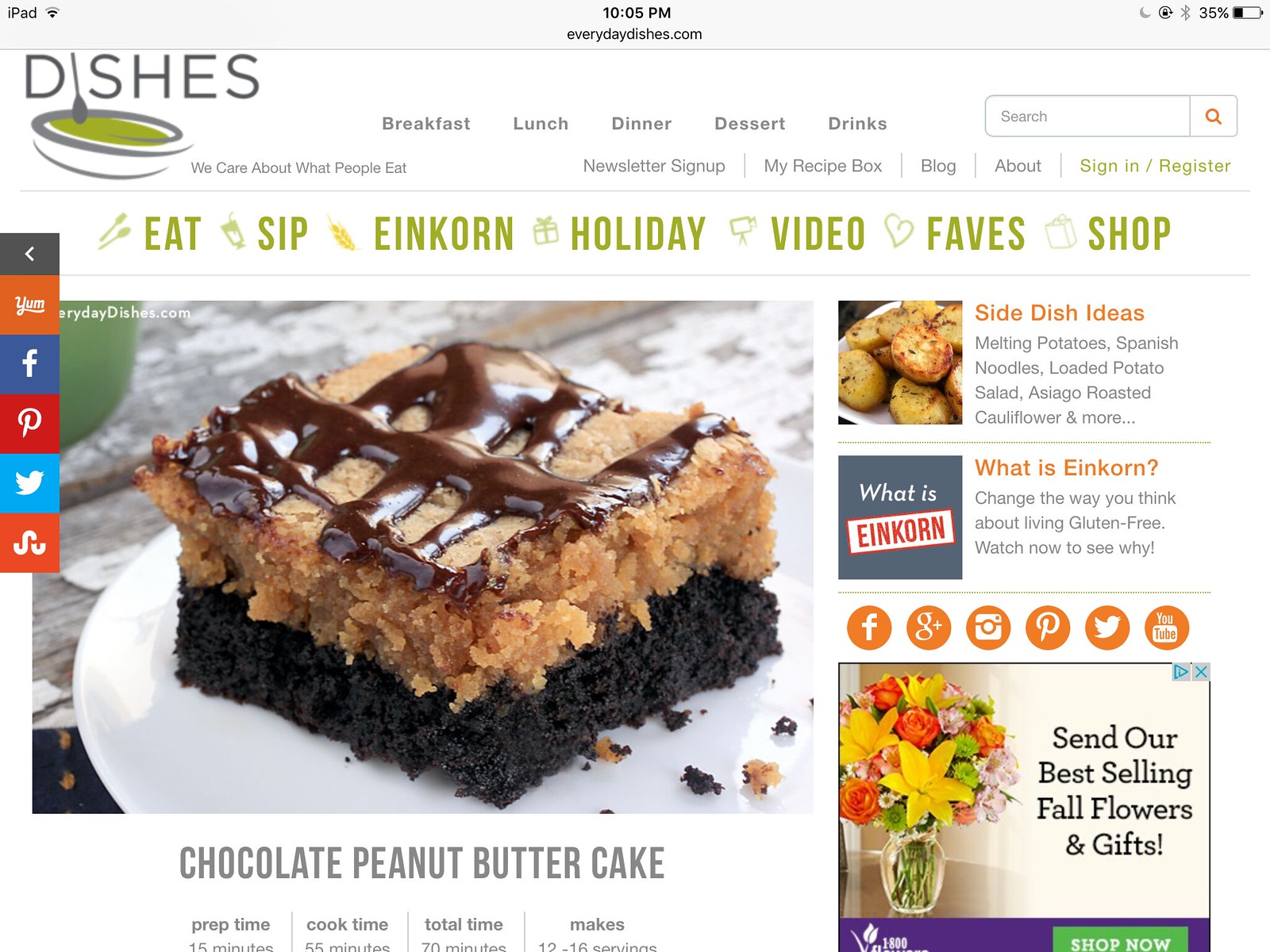The image is a detailed color screenshot of the recipe webpage everydaydishes.com in landscape orientation. At the top, the gray URL bar displays everydaydishes.com in black text. Immediately below, a banner features a logo on the top left with the word "DISHES" in black caps. A white bowl with green liquid and a spoon forming the letter 'I' in "DISHES" is part of the logo. To the right are labels for various categories including breakfast, lunch, dinner, dessert, and drinks, followed by large dark green text reading EAT, SIP, EINKORN, HOLIDAY, VIDEO, FAVES, and SHOP. A vertical row of social media icons is aligned on the left side of the page.

The central focus is on a large photograph of a Chocolate Peanut Butter Cake positioned slightly to the left, described as having a dark chocolate cake bottom with peanut butter crumblings on top, drizzled with chocolate syrup. The recipe details beneath the image specify a prep time of 15 minutes, cook time of 55 minutes, totaling 70 minutes, with a serving size of 12-16. On the right of the cake image is a small picture accompanied by the label SIDE DISH IDEAS, and a floral advertisement from 1-800-PRO-FLOWERS in the bottom right corner featuring a vase of colorful flowers. Additionally, the section WHAT IS EINKORN includes a corresponding color photograph of einkorn.

The webpage background is white, with a palette consisting of yellow, red, green, pink, brown, black, light green, and blue hues. The overall layout suggests a vibrant and accessible recipe website with an organized presentation of cooking ideas and advertisements.